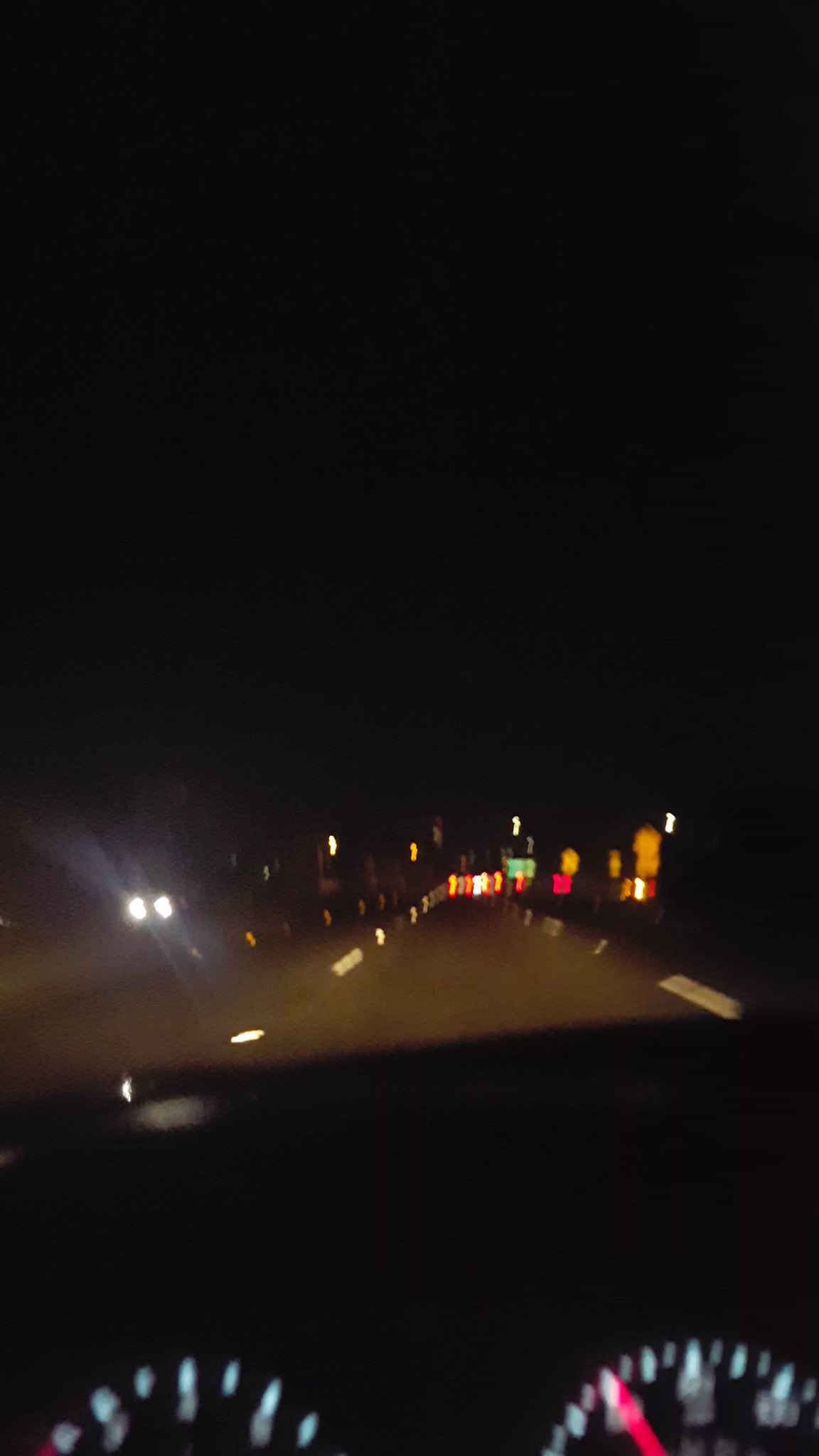This photograph, taken from the driver's seat of a car at night, captures a blurry and somewhat disorienting scene through the windshield. The sky dominates the upper two-thirds of the image, rendered as a deep, unrelieved black. The road ahead, faintly illuminated, shows a two-lane asphalt stretch with intermittent white dashes marking the lanes. To the left, blurry white headlights from oncoming traffic create glowing lines, characteristic of long-exposure night photography. The dashboard, shrouded in darkness, displays the top halves of illuminated speedometer and gas meter, featuring white numbers and letters on a black background, along with a prominent red needle on the speedometer. Reflective road signs and markers sporadically appear, though their details are muddled into yellow and black blurs. Small spots of green lights and other red and white lights add to the nighttime ambiance. Overall, the image's exposure is poorly adjusted, leading to numerous indistinct, brightly lit squares and rectangles that might be taillights or roadside signs, giving a sense of speed and movement. The vehicle appears to be driving on the right side of the road, suggesting an American setting.